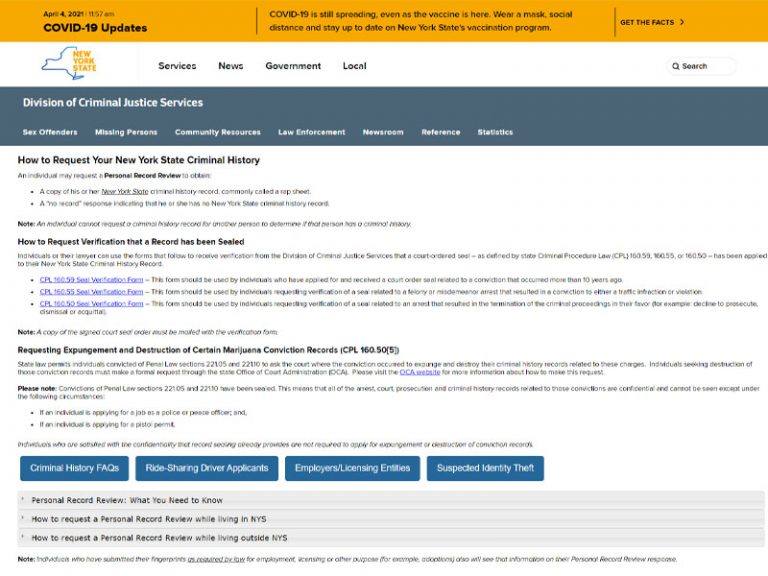**Detailed Caption:**

The image depicts a webpage from the New York State website providing COVID-19 updates dated April 4th, 2021, at 11:57 a.m. The upper section of the page features a prominent orange box with crucial information in black text: "April 4th, 2021, 11:57 a.m. COVID-19 Updates. COVID-19 is still spreading even as the vaccine is here. Wear a mask, social distance, and stay up to date on New York State's vaccination program." To the right of this message, there is a call to action with the text "Get the facts."

Situated below, on the left side, is an infographic specific to New York State. It includes the state's name in gold lettering and a blue outline of the state itself. Adjacent to the map are various navigation options including "Services," "News," "Government," "Local," and "Search."

Further down, the webpage provides detailed information related to the Division of Criminal Justice Services. This section is set against a dark blue/slate gray background with white text and includes headings for "Sex Offenders," "Missing Persons," "Community Resources," "Law Enforcement," "Newsroom," and "Reference and Statistics." 

Underneath, the section "How to request your New York State criminal history" includes instructions and options for requesting a verification of a sealed record, with several hyperlinks in blue text. Additionally, it outlines the process for "Requesting expungement and destruction of certain marijuana conviction records," referencing CPL 160.50/5 and the method on how to proceed.

At the bottom, there are blue buttons for various actions including "Criminal History Facts," "Ride Sharing Driver Applicants," "Employee Licensing and Titles," and "Suspected Identity Theft." Below these buttons is a dropdown menu with multiple options for managing personal records.